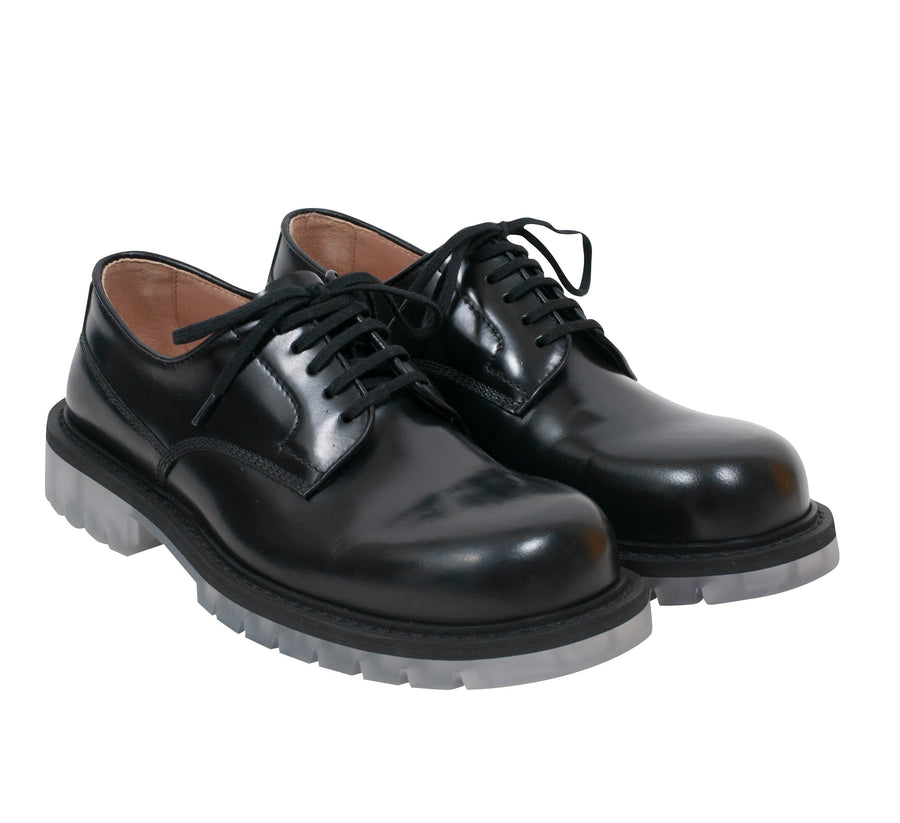The image showcases a pair of black, highly polished dress shoes that exude a vintage yet modern aesthetic, reminiscent of classic men's loafers. The shoes feature sleek black faux leather exteriors, complemented by thin black laces tied in neat bows. The interiors are lined with tan-colored material, and the shoes appear meticulously maintained, glistening as if freshly polished. What sets them apart is a distinctive platform sole, a frosted clear or light gray in hue, adding a unique touch to their otherwise traditional design. These shoes are positioned diagonally across a white background, from the upper left to the lower right, with the toes pointing to the right side of the image. They present a notable contradiction with their moderate heel, akin to those found on boots, enhancing the shoes' distinctive blend of styles.